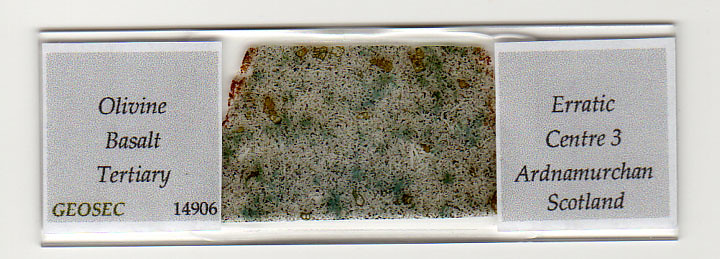The image depicts a rectangular glass slide, approximately six inches wide and two inches tall, framed by a light gray border. On the left side of the slide, there is a gray square label with black print reading "Olivine Faisal Tertiary." In the lower left corner of this square, green text spells out "Geosec", while the number "14906" is printed in black in the lower right corner. In the center of the slide, there is a textured specimen that appears to be a slice of stone, featuring a mix of green, white, and brown patterns, likely indicative of a mineral or geological sample. On the right side, another gray square label reads "Erratic Center 3, Ardenham Merchant, Scotland" in black print. The differing descriptions clarify the intricate details of the slide, emphasizing the characteristics and labeling of the specimen.